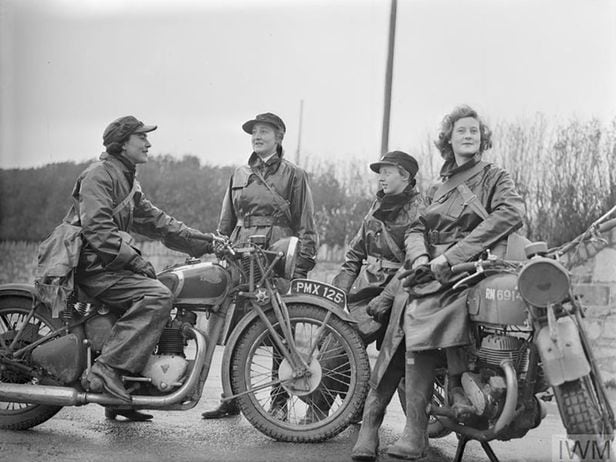This black and white vintage photograph, likely from the 1930s or 1940s, depicts four women with motorcycles on a wet street. The motorcycles display the identifiers "PMX125" and "RN6914," suggesting military or early generation models potentially from the WWII era. The woman on the left sports short hair, a hat, and a crossbody bag, and she stands beside her motorcycle, smiling and engaging with the others. Adjacent to her, another woman with longer hair leans against her motorcycle, wearing a long leather coat and distinctive cowboy boots. The women are uniformly clad in leather jackets resembling military or messenger attire. The background features dark trees, two large poles, and a gray sky, adding to the scene's historical ambiance.